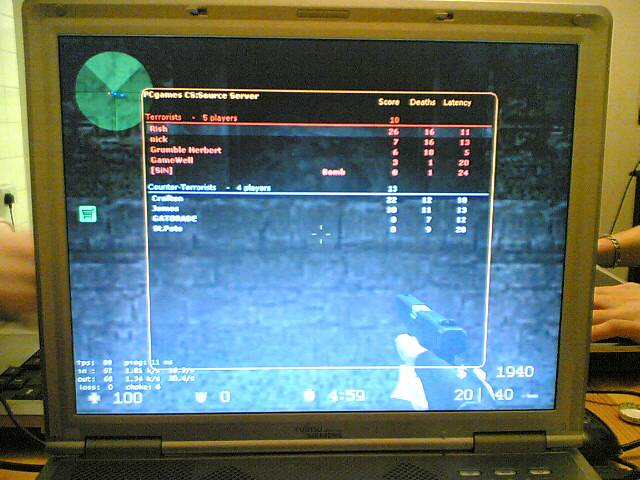This is a detailed close-up image of an active laptop screen. The laptop, encased in a sleek gray finish, shows only a portion of its bottom edge. The screen is illuminated, revealing a first-person shooter video game in progress. In the upper left-hand corner, there is a heads-up display (HUD) with a map, iconic to many first-person shooters. The in-game display indicates that the game has just concluded, transitioning to the end screen. In the lower right-hand corner, two hands gripping a gun are visible, characteristic of the first-person perspective. The background is slightly blurred, but elements of the game's environment can still be discerned.